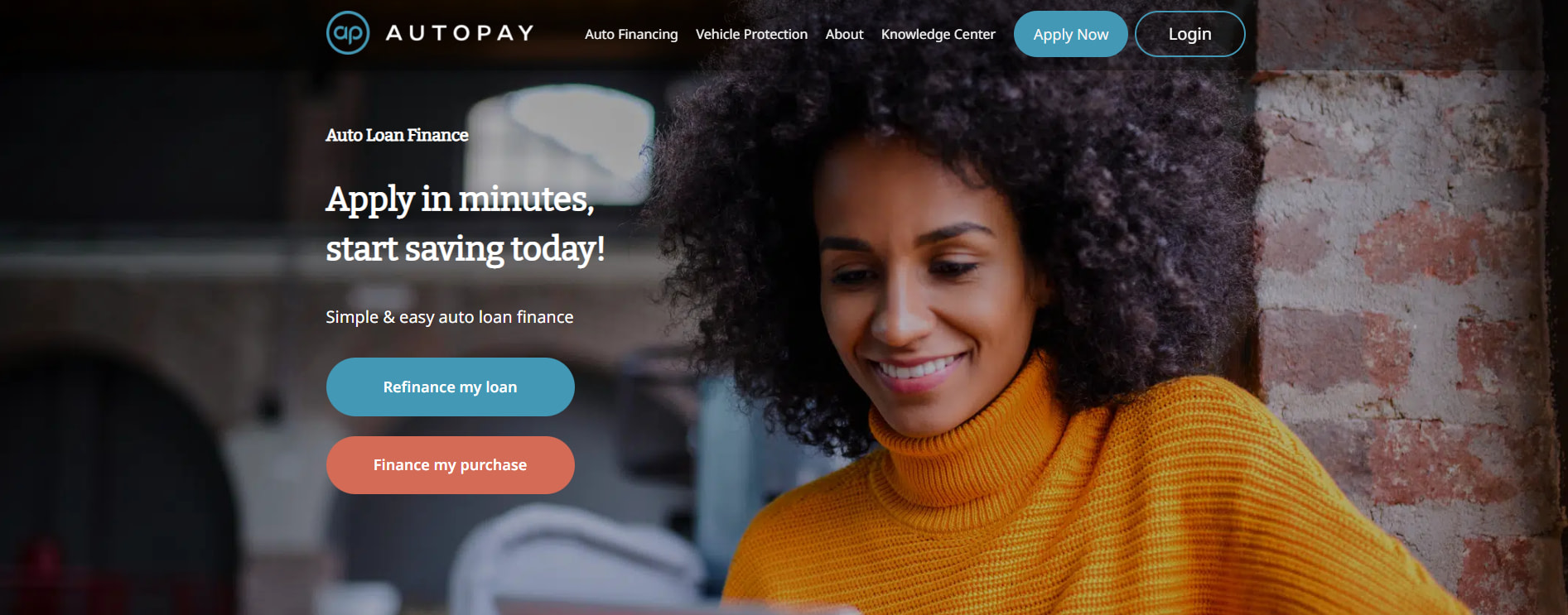This image resembles a promotional banner typically seen on major retail websites such as Target or Walmart. The background on the right side features a red and brown brick wall. In the foreground, there's a woman with curly, kinky black hair and brown skin, smiling warmly. She is dressed in a bright, mustard-yellow turtleneck shirt and appears to be interacting with a computer or tablet, which is partially visible at the bottom of the image.

The top left section of the image contains a series of navigational links in white text, including "Auto Pay," "Auto Financing," "Vehicle Protection," "About," and "Knowledge Center." Adjacent to these links, there is a teal oval button with white text that reads "Apply Now," and nearby, another oval outlined in teal with white text that says "Log In."

Below this, the text reads: 
- "Auto Loan Finance" in bold.
- "Apply in minutes" with "A" capitalized.
- "Start saving today!" followed by an exclamation point.
- "Simple, easy auto loan financing" with a hand symbol placed next to it.

Towards the bottom, there are two oval buttons:
- The first oval is teal with white text that says "Refinance My Loan."
- The second oval is a light red color with white text that reads "Finance My Purchase," with "F" capitalized.

Overall, the banner is designed to promote auto loan financing options, highlighting ease and convenience for potential customers.